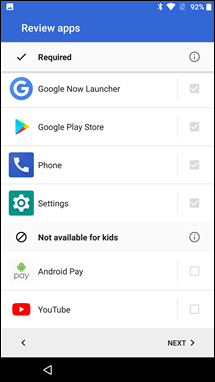A detailed screenshot of a smartphone in landscape mode showcases various settings and app reviews. The phone's status bar indicates that Bluetooth and Wi-Fi are enabled, the battery is at 92%, but there is no cellular signal or SIM card inserted. Dominating the upper section of the screen is a blue bar with white text reading "Review Apps." Directly beneath this bar, a list of applications is displayed with corresponding checkmarks indicating whether they are selected or not. 

The checked applications include:
- Google Now Launcher
- Google Play Store (icon: stylized play arrow)
- Phone Settings (icon: gear)

Apps that are not checked, indicating they are possibly restricted, are:
- Android Pay
- YouTube (icon: play button)

This suggests that the phone is likely set up for parental control or a similar purpose.

Navigation buttons for "Back" and "Next" are present, with the "Back" button also situated at the bottom of the screen. Each listed app is accompanied by a corresponding icon for easy identification. The overall background of the screen is white, creating a clean and straightforward interface for app review and selection.